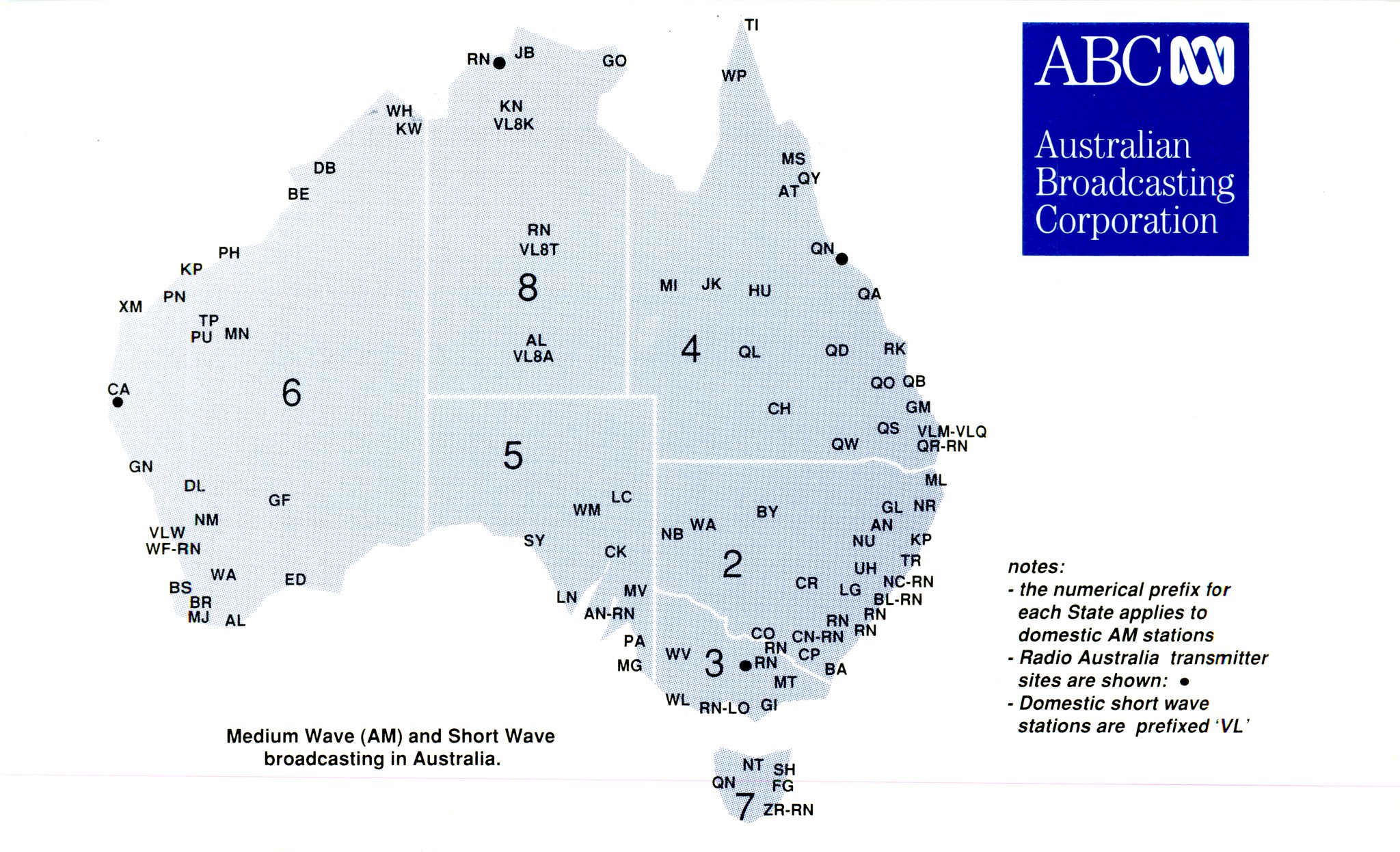The image depicts a detailed map of Australia, primarily in grey against a white background, showcasing various regions or states, each labeled with different numerical prefixes (such as 2, 3, 4, 5, 6, 7, and 8) to indicate domestic AM radio station frequencies and broadcast sites. In the upper right corner, a blue square features the white letters "ABC" along with a stylized swirl logo and the text "Australian Broadcasting Corporation" below it. Additional notes on the map explain that the numerical prefixes apply to domestic AM stations, and indicate transmitter sites for Radio Australia. The map also points out that domestic shortwave stations are prefixed with "VL." The entire layout seems to include details about medium wave AM and shortwave broadcasting locations across Australia, suggesting that the image might have been scanned from a printed source.